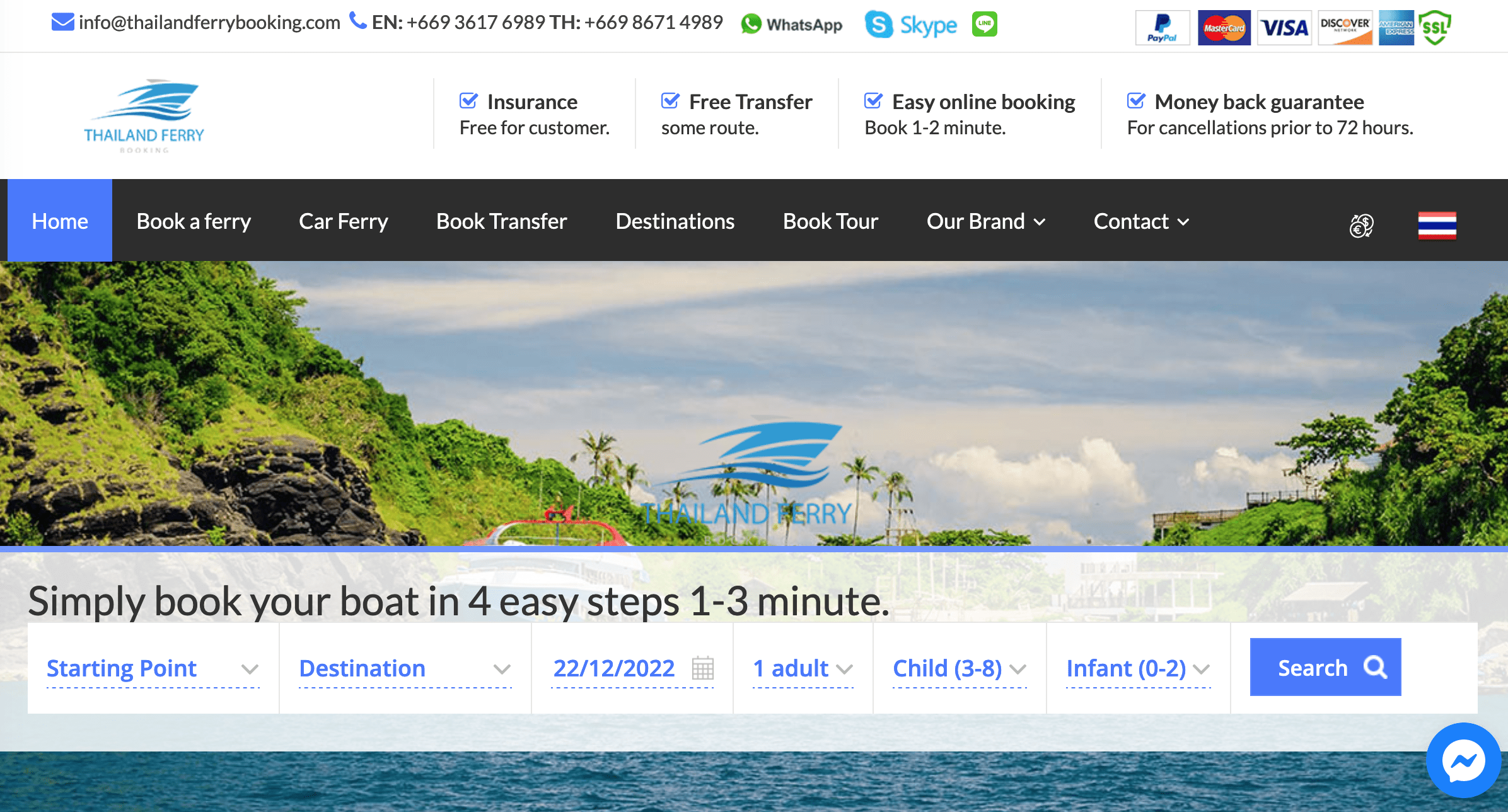This screenshot captures a comprehensive view of the Thailand Ferry Booking website. At the very top, the site's contact information is prominently displayed, including email info@thailandferrybooking.com, and phone numbers for English-speaking (+66 9-3617-6989) and Thai-speaking (+66 9-8671-4989) customers. Icon links to WhatsApp, Skype, PayPal, Mastercard, Visa, Discover, American Express, and SSL ensure a multitude of communication and payment options.

Beneath this section, a simple yet illustrative line drawing of a boat navigating waves appears. Below it, the text "Thailand Ferry Booking" is bold and clear. The service highlights are organized neatly: "Insurance, free for customer," "Free transfer some route," "Easy online booking, book 1-2 minute," and "Money back guarantee for cancellations prior to 72 hours."

Next is a black menu bar with white lettering, except for the "Home" section which is outlined in blue to show it is selected. The menu options are "Book a ferry," "Car ferry," "Book transfer," "Destinations," "Book tour," "Our brand," and "Contact." At the right end of the menu bar, images of a euro coin overlapping a dollar coin are displayed, along with a flag featuring horizontal stripes of red, white, blue, white, and red.

The main image on the webpage is a serene scene showing emerald green rocky hills on the left, distant palm trees, and additional trees and buildings to the right. Overhead, the sky is cloaked in clouds, giving a calm ambiance. The faint silhouette of the top part of a boat can be seen in the distance.

A bottom banner simplifies the booking process with the message, "Book your boat in 4 easy steps, 1-3 minute." The user is prompted to enter details such as starting point, destination, date (22-12-2022), and the number of passengers (one adult, one child aged 3-8, and one infant aged 0-2), with the search function conveniently located.